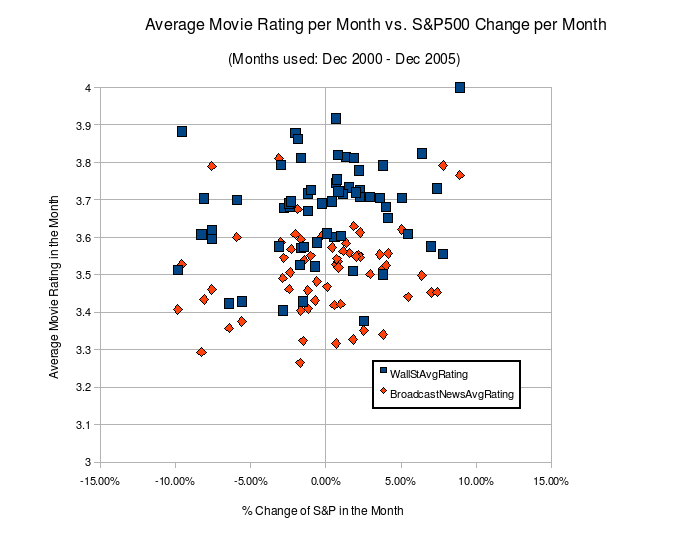The image is a detailed graph titled "Average Movie Rating per Month vs. S&P 500 Change per Month," utilizing data from December 2000 to December 2005. The Y-axis represents the average movie rating per month, with a range from 3 to 4. The X-axis illustrates the percentage change in the S&P 500 per month, spanning from -15% to 15% in 5% increments. 

The graph plots data points using blue squares for Wall Street's average movie ratings and orange diamonds for broadcast news' average movie ratings. Both sets of data points are predominantly clustered around the center, where the S&P 500 change is near 0%, and the average movie ratings range approximately from 3.5 to 3.7. There are no significant data points at the extremes of -15% or 15% S&P 500 change. A few outliers exist, including a point reaching an average movie rating of 4.

Overall, the chart maintains a concentrated central distribution, with most points indicating little correlation between extreme S&P changes and movie ratings, necessitating a closer analysis for further insights.